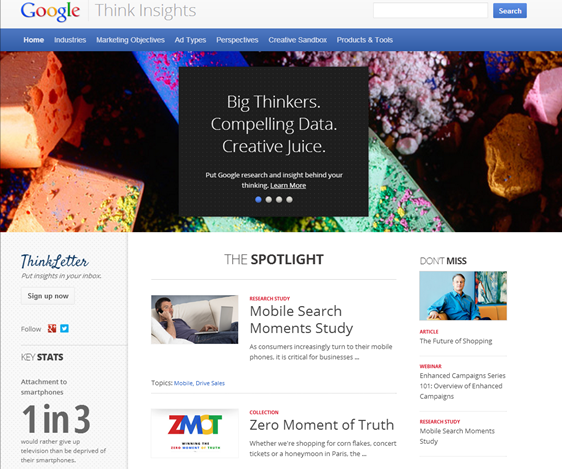The image features a webpage with a grey bar at the top, displaying the multicolored Google logo (blue, red, yellow, blue, green, red) next to the phrase "Think Insights" in grey text. Below this, a search bar occupies the center, flanked by a blue "Search" button with white text on the right. Underneath, there is additional white text on a blue background.

On the left-hand side, a vertical menu lists the following options: Home, Industries, Marketing Objectives, Ad Type, Perspective, Quality Sandbox, Products and Tools. The main content area has a dark background with vibrant elements in white, blue, green, and red hues. Centrally, a black box with white text reads: "Big Thinkers, Compelling Data, Creative Juice. Put Google Research and Insight Behind Your Thinking." Below this phrase is an underscored "Learn More" link next to four dots, with the first dot colored blue and the other three white.

The central section of the image shows a spotlight effect highlighting a person lying on a couch with their cell phone in hand, looking at a MacBook. Adjacent text reads "Mobile Search Movement Study," referring to an investigation of mobile search behaviors. Further along to the right, the term "ZMOT" is explained as "Zero Moment of Truth," an acronym Google proposes for a crucial decision-making point in the customer journey.

In the rightmost part of the webpage, a "Don't Miss" section draws attention with an image of a person sitting on a yellow couch wearing a blue shirt, with an expression that suggests tension or discomfort.